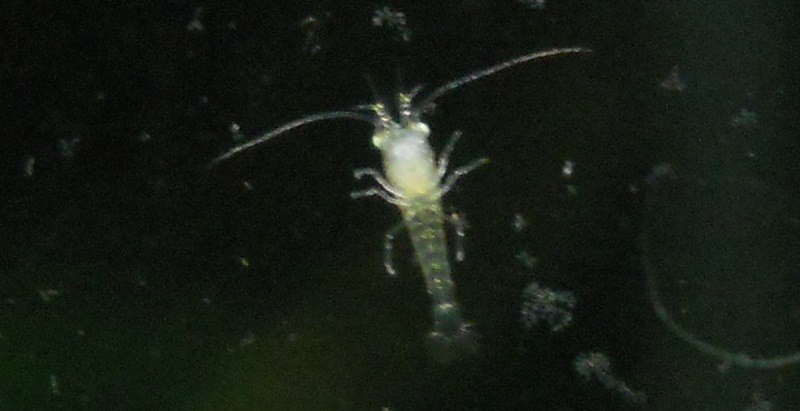In this very blurry and heavily zoomed-in image, the primary subject appears to be a small sea creature, likely a crayfish or a tiny crustacean, possibly under a microscope. The creature is positioned against a dark, almost black background, scattered with white, blurry specks that resemble debris or small particles, which could be indicative of a microscope slide preparation. The crayfish itself is somewhat translucent with a predominantly greenish body, white head likely exaggerated by a camera flash, and intricate black stripes along its form. Its tail has a distinct black tip, and from the underside, the tail appears translucent. It features six legs and astonishingly long antennas, extending beyond the length of its body. The creature’s anatomical details suggest it might be illuminated from below, further contributing to its otherworldly, translucent appearance in the dark surrounding. Additionally, there seems to be some speculation of a tentacle-like structure in the background alongside other particles.